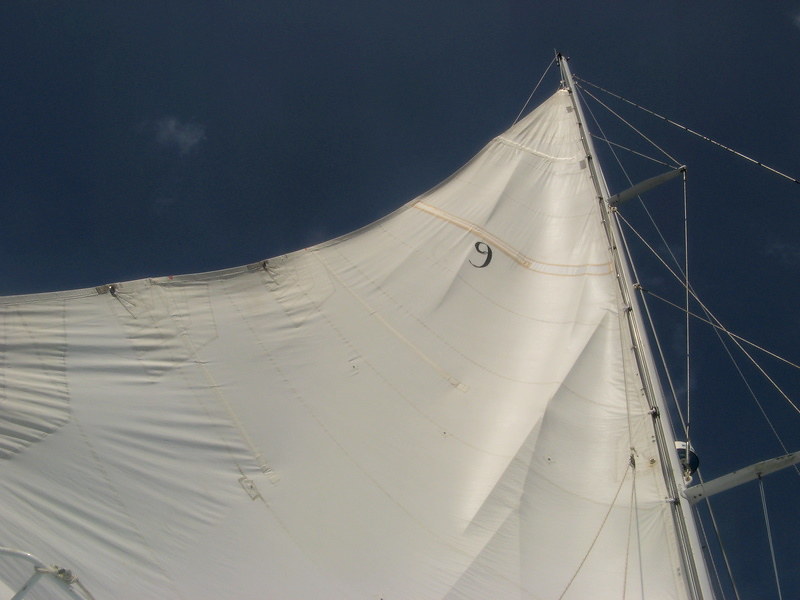A large white sail, marked with the number nine near its top, dominates this photograph. The sail, which features visible stretch marks and some brownish, off-colored patches indicating wear, is part of a sailing boat or yacht. The photograph, taken from a ground-up perspective, showcases the mast and an array of ropes, rigging, and wires supporting the sail. The background reveals a dark, navy blue sky with a hint of a small, puffy white cloud. Despite the seemingly illuminated environment, the sun is not visible, and no water can be seen. The image captures the stretched sail in detail, highlighting the network of lines and the overall landscape format of the scene.